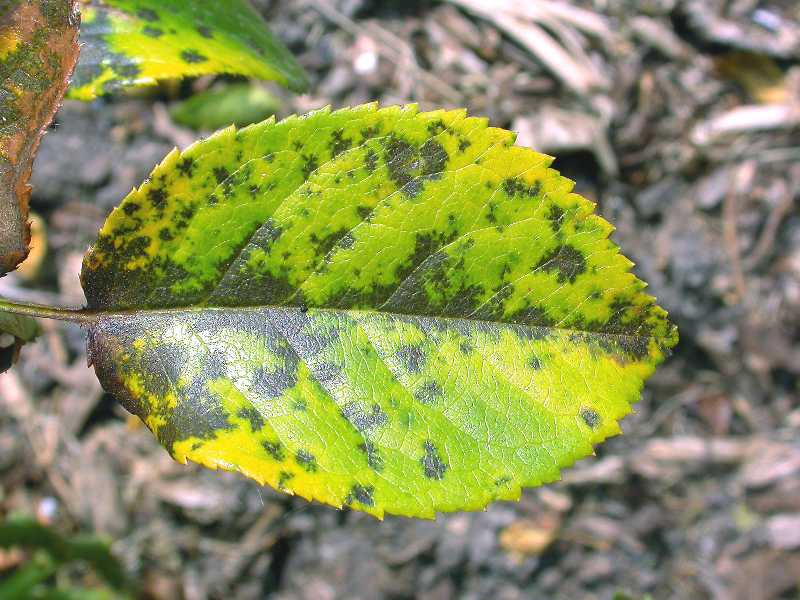This detailed photograph focuses on a single, striking leaf set against a blurred background, likely of dead brush or brown ground. The leaf is vibrantly lit and exhibits a neon to lime green color that stands out with an almost neon brightness. Complementing this vivid green are splotches of dark, metallic gray and occasional brown spots, predominantly centered on the leaf but also scattered towards the top and bottom edges. The leaf is oval-shaped with distinctly serrated, ridged edges running along its entire perimeter. In the background, other leaves are visibly turning brown, with one appearing entirely browned. A partial view of the stem and a small branch in the top left corner suggests the leaf might be attached to a larger plant. Despite the background blur, the image is of high quality, clearly capturing the intricate details and contrasting colors of the leaf.